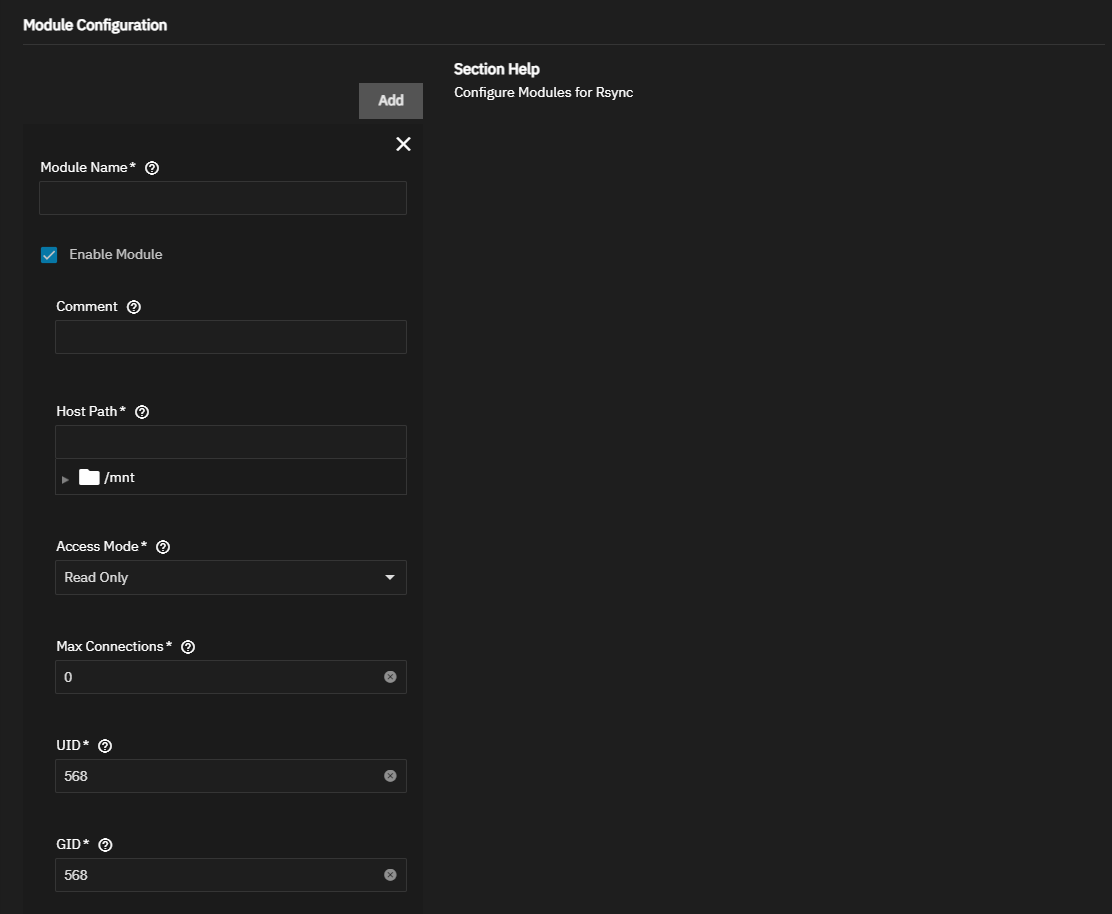This image showcases a software interface set in landscape mode. The majority of the screen is black, with text and interface elements providing specific functions. In the upper left-hand corner, in white text, is the title "Module Configuration." Below this title, a light gray line extends horizontally all the way to the right edge of the screen.

The interface is divided into two main columns. 

**Right Column:**
- The header reads: "Section help configure modules for RSYNC."
- The remainder of this column is blank, leaving a large black space.

**Left Column:**
- At the top of this column is a gray "Add" button.
- Beneath it is a white "X" icon.
- Below the icons, text fields and labels align sequentially: 
  - "Module name *" followed by a help icon represented by a question mark within a circle. This field allows the user to input the name of the module.
  - A blue check mark is present to enable the module.
  - Text fields for "Comments," "Host path" (with an example "/mnt" and a folder icon), and "Access mode," which is set to "Read-only."
  - Settings fields include "Maximum connections: 0," "UID: 568," and "GID: 568."

This screen is clearly intended for an individual, likely using a laptop, who is configuring a module within the RSYNC utility, specifying details such as the module name, comments, host path, and various access settings.